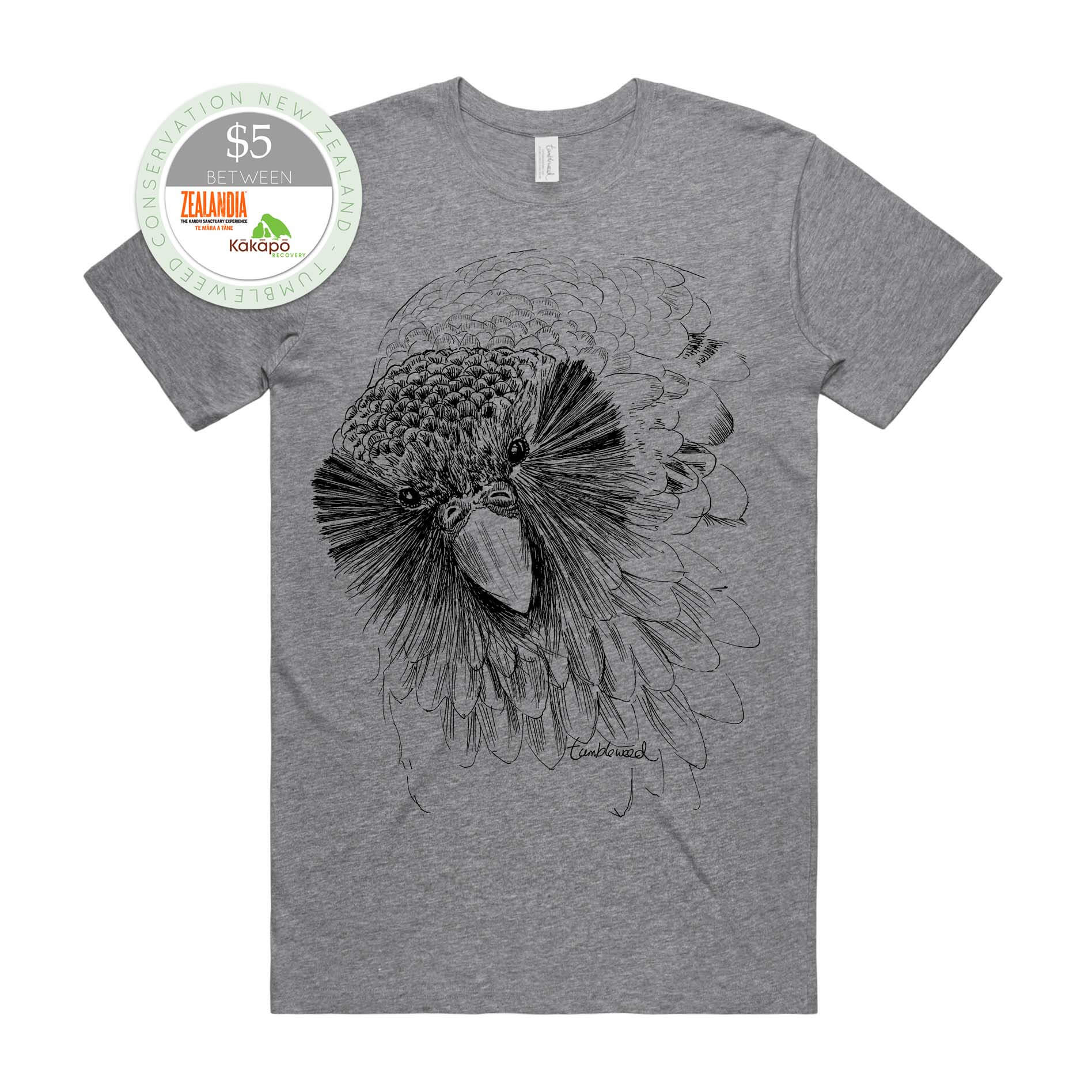This image showcases a mock-up of a gray, short-sleeved t-shirt laid flat against a solid white background, which dominates the majority of the frame. The t-shirt features a detailed black and white graphic of a bird prominently displayed in the center, highlighting the bird's face and feathers with intricate detail. Positioned on the top left shoulder is a circular label with a green outline, bearing the text "Tumbleweed Conservation New Zealand," and "$5" placed between the logos of Zealandia and Kakapo. Additionally, there is a white tag attached to the collar of the shirt. The overall presentation emphasizes both the aesthetic and branding elements of the t-shirt, giving it a clean and professional appearance.